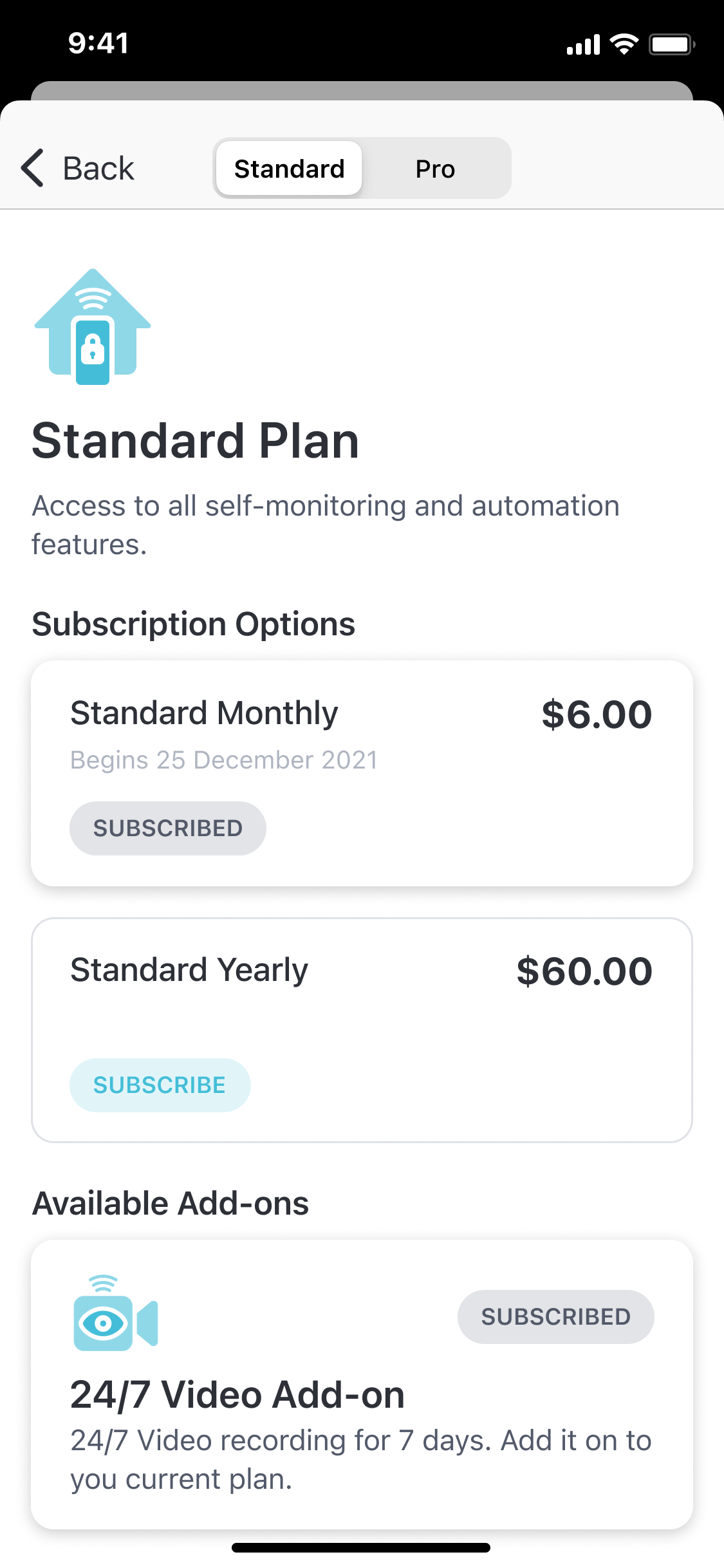This is a screenshot of a phone's display taken at 9:41 AM, showing a fully charged battery and a strong Wi-Fi connection. The screen shows subscription details for a service under the "Standard Plan." Highlighted in blue above the plan options is a home icon, indicating the subscription tier. The user is subscribed to two plans: a "Standard Monthly" plan costing $6 and starting on December 25, 2021, and a "Standard Yearly" plan priced at $60. Below these plans, there are available add-ons, including a "24/7 Video Add-on" with a blue camera icon above it and a gray "Subscribe" button next to it. The layout provides clear options for the user's current plan and additional features they can subscribe to.